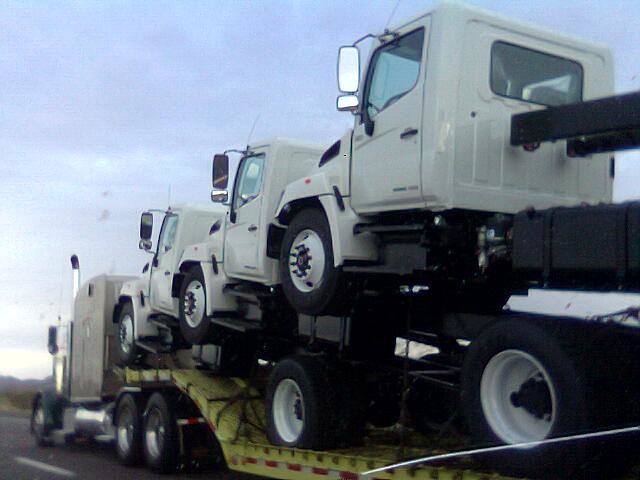The photograph captures an intriguing scene of a tan semi-tractor with a silver fuel tank and exhaust pipe hauling a neon yellow flatbed trailer along a tarred highway, delineated by a white line on the left side. Against the backdrop of a partly cloudy blue sky, tinged with the hues of a setting sun, the semi is transporting three identical white semi-tractors. These tractors are precisely stacked: the first is perched on the gooseneck of the trailer, the second on the flatbed of the first, and the third atop the second. Each of these white tractors boasts black frames, distinct driver's cabs, and a black section where a trailer would typically connect. They are equipped with white center wheels, black tires, and large rectangular mirrors accompanied by smaller square ones beneath. In the distance, a horizon line reveals a mountainous range with modest greenery, adding depth to the scene. The reflective lights along the edge of the yellow flatbed glint subtly, harmonizing with the dimming light of the impending dusk.